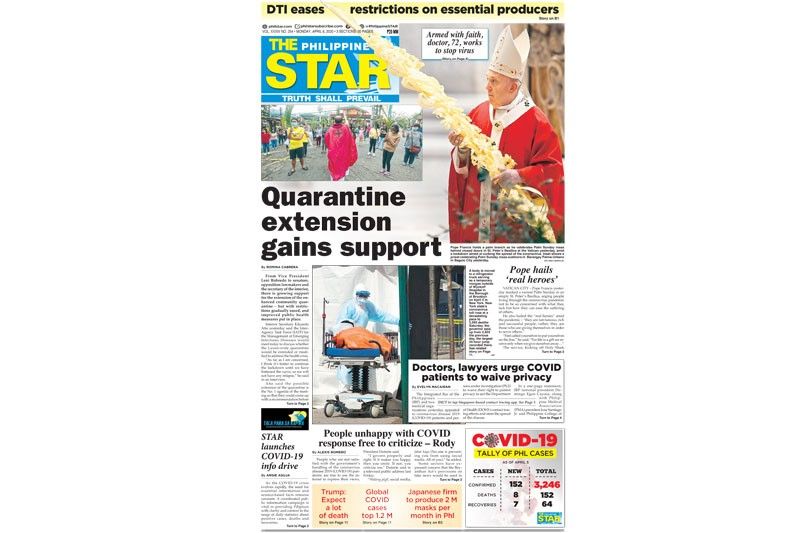The image depicts a cluttered front page of the Philippine Star newspaper, clearly captured from a physical copy. The top section features a yellow horizontal strip with the headline "DTI eases restrictions on essential producers," though the date is too small to be legible. 

Beneath the newspaper's header, which reads "Philippine Star" accompanied by the motto "Truth Shall Prevail," there are six breakout boxes for various news stories. Each box contains both text and visuals, contributing to the visually busy layout:

1. **Main Story: "Quarantine Extension Gained Support"**
   - Visual: An image of a march with people protesting on the streets.
   
2. **"Armed with Faith"**
   - Visual: A photograph of the Pope in full papal regalia, including his white cap.
   - Subheading: "Dr. 72 works to stop virus."
   - Subheading: "Pope hails real heroes."

3. **"Doctors, Lawyers Urge COVID Patients to Waive Privacy"**
   - Visual: A man in a full white hazmat suit wheeling a patient on a gurney out of what appears to be a hospital room or quarantine space.

4. **"People Unhappy with COVID Response Free to Criticize – Brody"**
   - Visual: A graphic displaying the COVID-19 tally of Philippine cases.

5. **"Star Launches COVID-19 InfoDrive"**
   - This story does not appear to have an associated image.

Below these feature articles, the page contains dense sections of fine print, presumably the main news stories and accompanying details in very small text. The design is vibrant, filled with numerous colors and images, making the page appear overwhelmingly busy and cluttered.